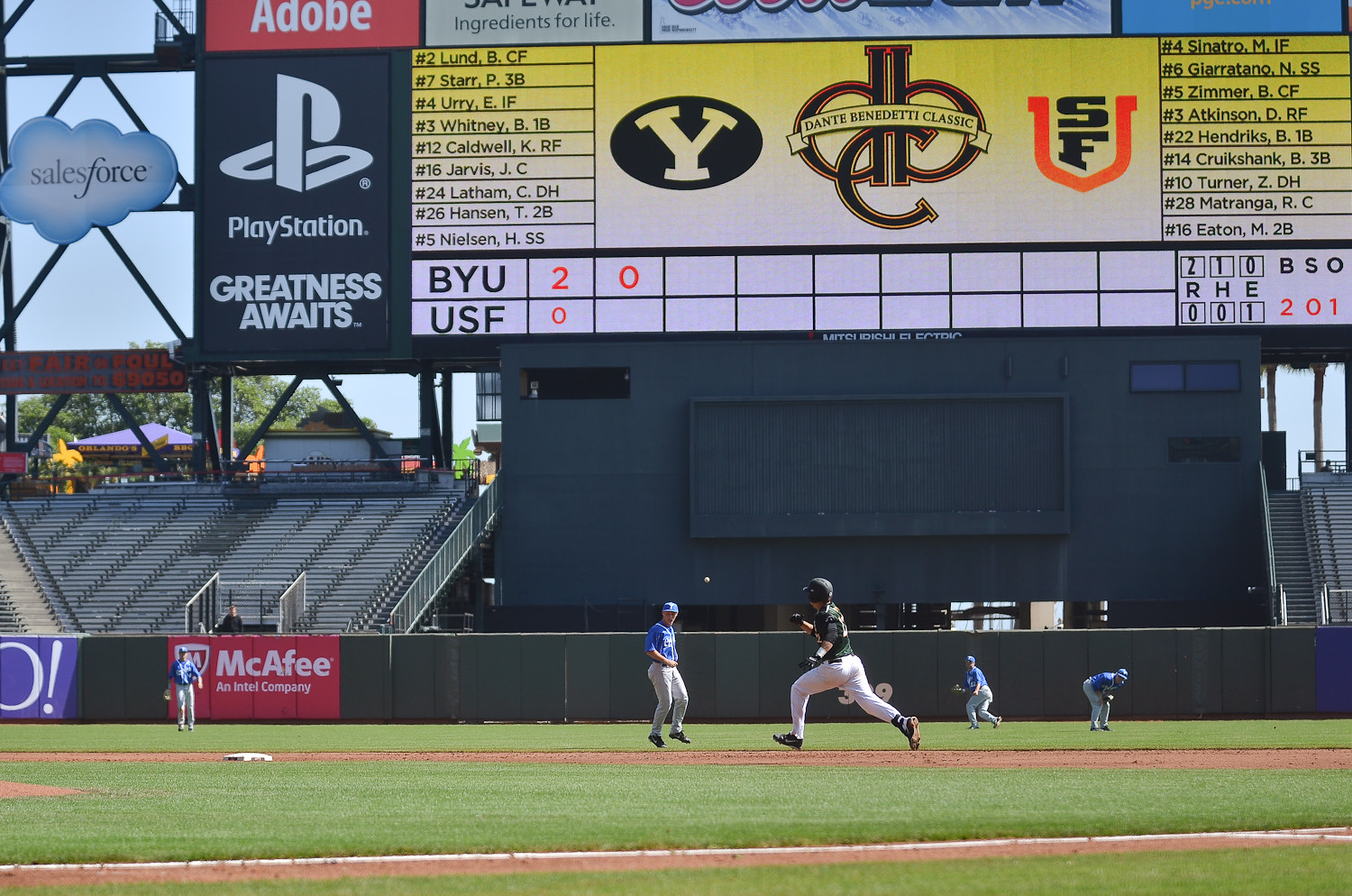The image captures a vibrant college baseball game between BYU and USF, viewed from ground level in landscape orientation. The green expanse of the baseball field contrasts with the brown dirt around the bases. A lively scene unfolds as a player in a green shirt, white pants, gloves, and a hat—possibly a batting helmet—runs toward the next base. Opposing him, several players in blue jerseys and hats are scattered across the outfield, poised to make a play. The empty stands tower above the field, leading up to a gigantic scoreboard that dominates the background. The scoreboard displays the score, with BYU leading 2-0, alongside a plethora of sponsor logos such as PlayStation, Adobe, and Salesforce. Additional ads line the wall behind the field, blending into the realistic and bustling atmosphere of the game.